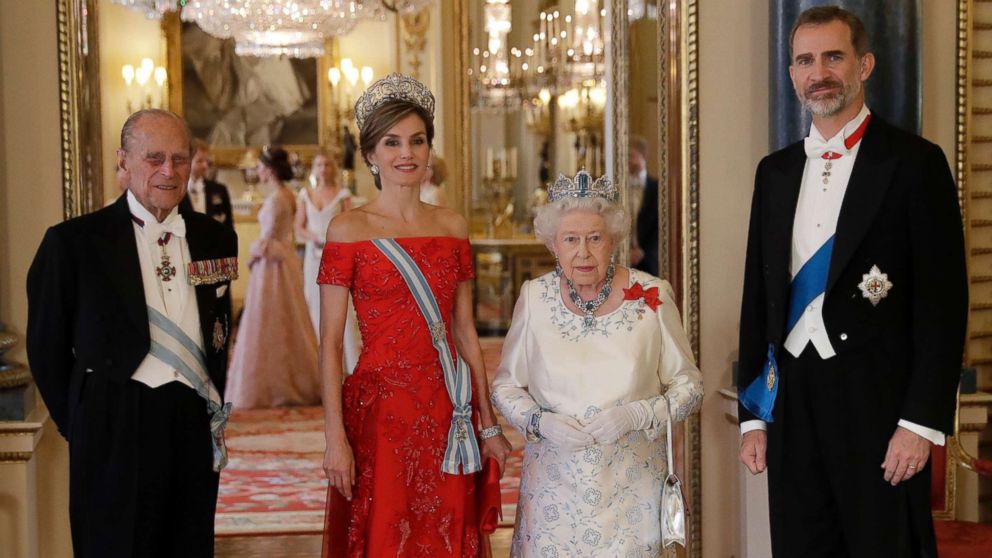The photograph depicts an elegant scene featuring prominent members of the British and Spanish royal families, set in what appears to be the opulent interiors of Buckingham Palace, marked by chandeliers, mirrors, and ornate decor. In the center of the image stands Queen Elizabeth II in her advanced age, adorned in a white embroidered floral dress, white gloves, and holding a silver handbag. Her attire is complemented by a majestic and ornate crown featuring blue sapphires or blue diamonds, and a necklace with similarly hued gemstones. To her right is Prince Philip, Duke of Edinburgh, dressed in a black tuxedo with a white shirt. He dons a blue sash, a red medallion around his neck, and a decorated star-shaped badge on his chest. On Queen Elizabeth's left stands what appears to be the Spanish Queen, dressed in an off-the-shoulder bright red gown with a light blue and white sash. She wears a tiara and glistening diamond earrings. Next to her is the Spanish King, characterized by his grey beard and advanced age, dressed in a classic tuxedo featuring a blue sash and a red collar. Observing the scene from the background, other royals such as Kate Middleton and Prince Harry are faintly visible, adding to the grandeur and historical significance of the captured moment.